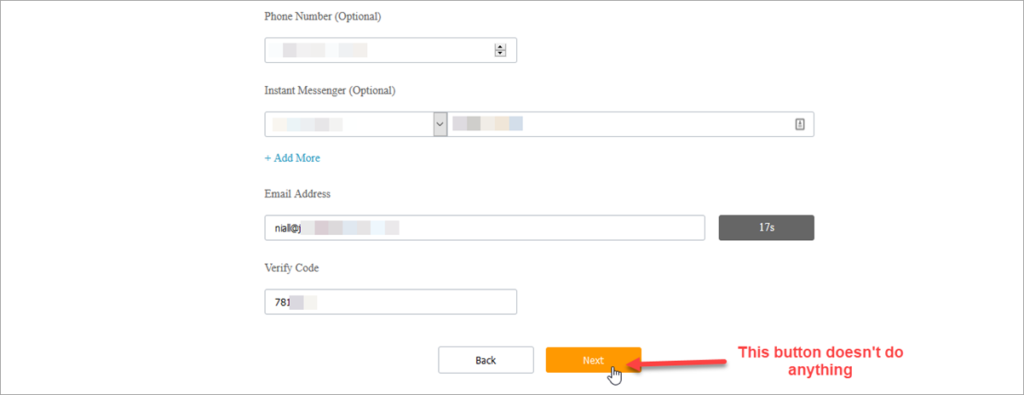The image features a form on a pristine white background, intricately outlined in gray. At the top, slightly left of center, the text "Phone Number" appears in bold black font, followed by the word "optional" in parentheses. Below this, there's a data entry field for typing in the phone number.

Further down, there's a section labeled "Instant Messenger," also with "optional" in parentheses. This is accompanied by a banner where the user can type a message. However, the content in this banner appears grayed out. Adjacent to it, another banner is visible, featuring little gray boxes that obscure the entered text. Directly beneath this section is a blue plus sign, with the phrase "Add More" in matching blue.

Below this, the form requests an "Email Address" in bold black text, followed by another data entry banner where an email address is partially typed but grayed out with gray boxes. On the right side of the form, there's a dark gray banner stating "17S," although its significance is unclear.

To the left again, the text "Verify Code" is shown with a corresponding entry banner below it. Here, the digits "781" are visible, but the remainder of the code is covered by gray boxes.

At the bottom, two prominent buttons stand out. The left button is outlined in black and labeled "Back," while the right button is a vibrant orange with the text "Next" in white. An illustration of a hand with a pointing finger, accompanied by a red arrow, directs attention to the orange "Next" button. Notably, a red warning beneath this button states, "This button doesn't do anything."